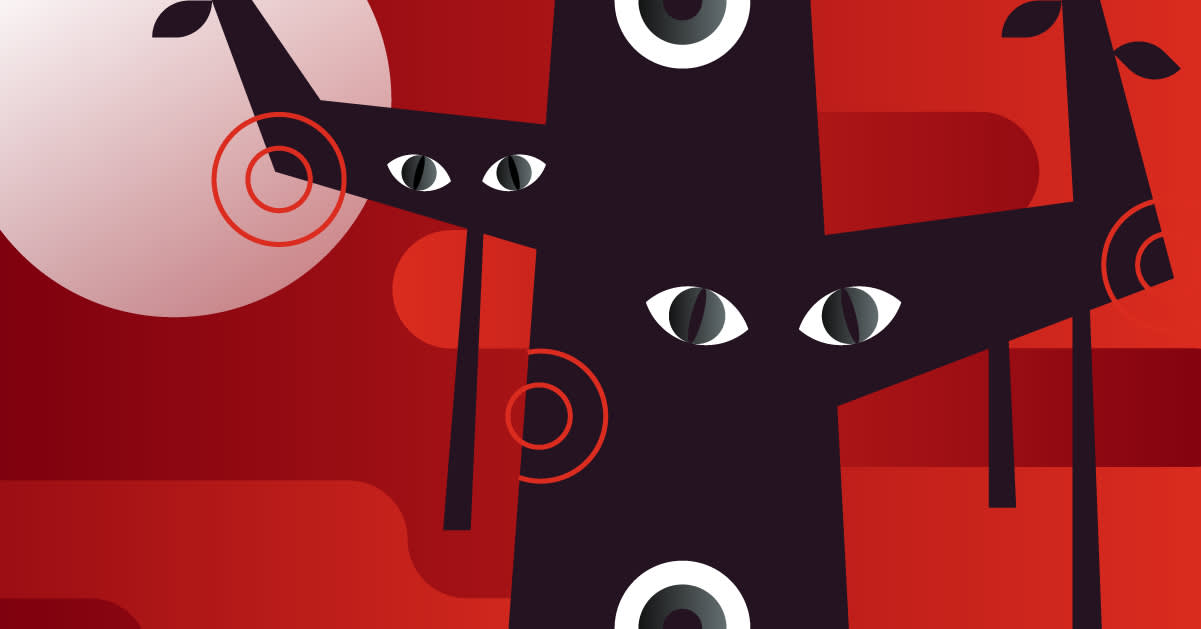The image is a modern, abstract depiction of a tree characterized by its unusual and evocative features. The tree, rendered in a dark gray to black shade, stands prominently against a vivid background of varying red and orange hues. It features two prominent branches that bend at the elbows and rise upwards, reminiscent of human arms. Unusually, the trunk and one of the branches are adorned with eyes—specifically, two pairs of eerie, cat-like eyes with gray pupils, peering out as if alive.

A pale pink orb, likely representing the moon or sun, is situated in the top left corner of the composition, enhancing the surreal ambiance. Scattered throughout the image are several red concentric circles that add to its abstract nature. The composition is minimalist in its use of straight lines and stark contrasts, creating a blend of unsettling and intriguing visual elements. The overall effect is a striking fusion of natural and unnatural motifs, leaving viewers to ponder the mysterious, animated-like scene.